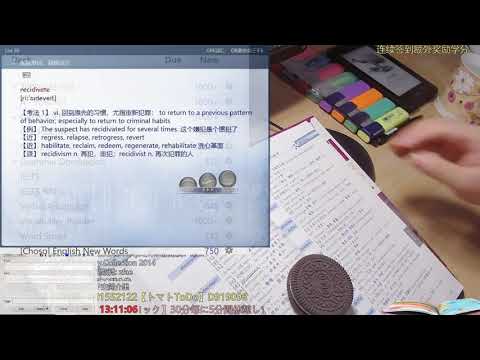The image captures a detailed scene on a brown wooden desk. In the foreground, there is an open notebook filled with both English and Asian characters, including phrases like "the suspect has recidivitated for several times, regressed, relapsed, retrogressed, revert," suggesting language study. An Oreo cookie rests atop the notebook. A motion-blurred hand hovers near the center right. Organized neatly on the desk are multicolored highlighters in yellow, teal, orange, purple, green, pink, and blue. Next to the highlighters is a black smartphone and a white mug adorned with a pink and yellow floral pattern. In the background, there's a computer screen displaying an email application with English and Chinese text, partially pixelated, and words like "choose a English new words." Additionally, the image shows a few scrolling times in red and Chinese characters. The bottom right of the screen features elements that resemble globes or marbles.